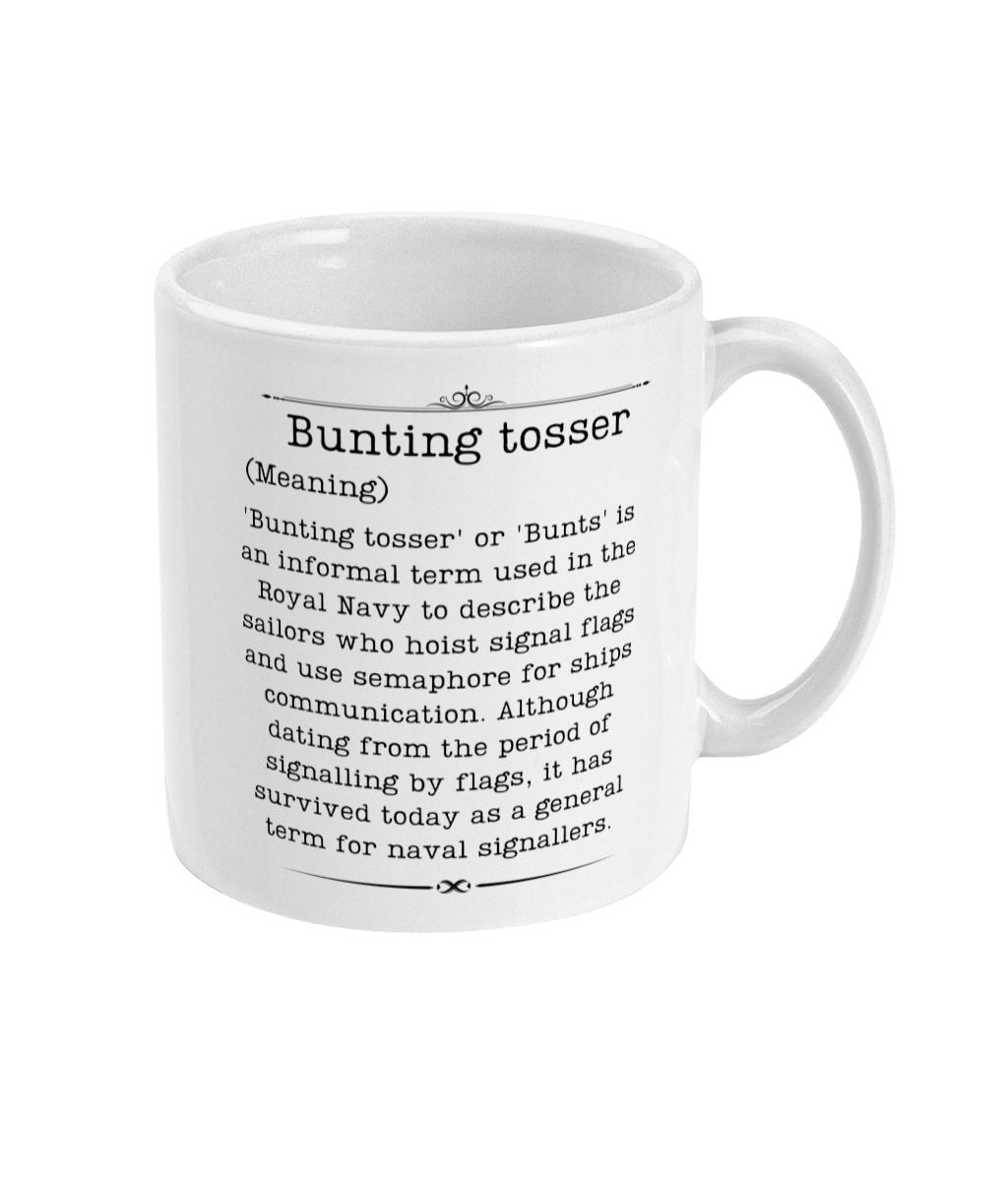In this close-up image of an ivory white ceramic coffee cup with a handle, the cup is prominently centered against a white background and features black text on its side. The text reads: "Bunting tosser," followed by a definition, "Bunting tosser, or bunts, is an informal term used in the Royal Navy to describe the sailors who hoist signal flags and use semaphore for ships' communication. Although dating from the period of signaling by flags, it has survived today as a general term for naval signalers." Decorative elements include black lines above and below the text, with the bottom line separated by an infinity symbol. The coffee cup is empty, and this minimalistic photograph emphasizes the detailed and historical description on the cup.